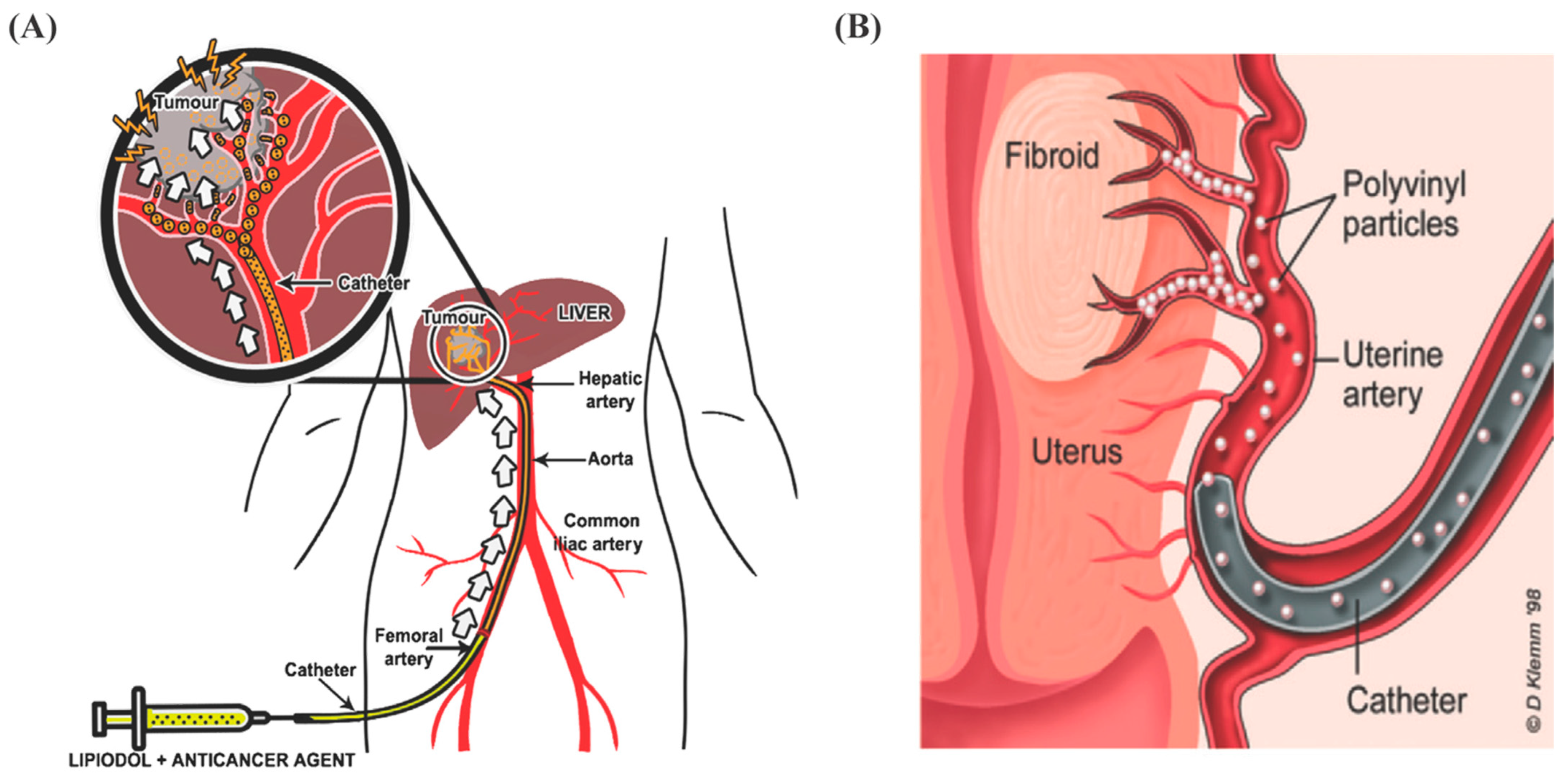This image features two anatomical diagrams labeled as "A" and "B" against a white background, designed for educational purposes in teaching anatomy and physiology. 

**Panel A** is situated on the left and presents a detailed depiction of the human liver. The liver is shown with a highlighted yellow area marked as a tumor. Several arteries are branching out from the liver, including the aorta (colored red), the hepatic artery, the common iliac artery, and the femoral artery, all clearly labeled. A yellow catheter is inserted into the femoral artery, connected to an injection device labeled "lipidol, anti-cancer agent." The catheter is shown delivering the medicinal agent towards the grey-colored tumor, with white arrows illustrating the flow direction. The tumor area is further magnified in the top left corner within a black-ringed red circle, providing an enlarged view of the catheter entering the tumor.

**Panel B** on the right shows the pelvic region, specifically focusing on female reproductive anatomy. This diagram uses pink and red hues to represent the uterus and associated structures. A central light pink circular area is labeled as a fibroid, located within the uterus. The uterine artery, depicted in red, branches out with the presence of white, pearl-like structures labeled as polyvinyl particles. These particles are being delivered through a grey catheter. Important anatomical structures such as the fibroid, the uterus, the uterine artery, and the polyvinyl particles are explicitly labeled for clarity.

Both panels, A and B, serve to illustrate the application of medical devices such as catheters in the treatment of tumors and fibroids, providing a clear and detailed educational reference. At the bottom right corner of the image, there is a watermark labeled "Copyright D. Clemmon 98".